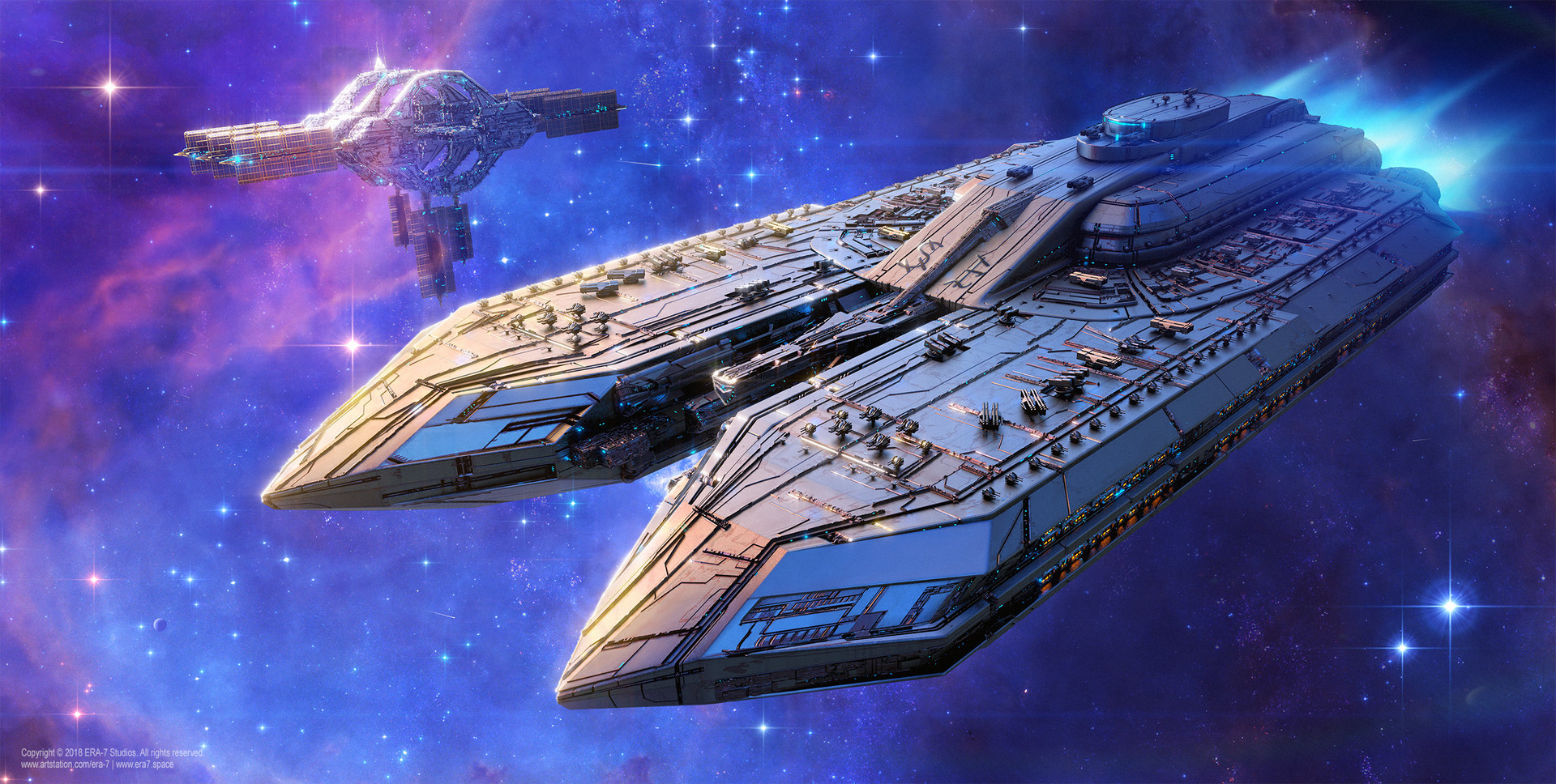The image is a highly detailed computer-generated science fiction illustration set against a vibrant blue and purple outer space background filled with cosmic dust and a multitude of bright stars. The central subject is a colossal spaceship composed of two arrow-like, three-dimensional shapes, reminiscent of picket fence stakes, fused together. This massive spacecraft features various elements attached to its surface, including blasters at the rear, a tall front section, and numerous guns positioned around a deck-like platform. In the middle section of the spaceship, there's a distinct inset area forming a gap between the two pointed front ends.

In the upper left corner of the image, a cross-shaped space station with prominent rings in its center is visible, adding to the sense of an extensive, inhabited galaxy. The spaceship is oriented with its pointed ends directed towards the bottom left of the frame. The bottom left of the image clearly displays a copyright notice in white lettering: "Copyright 2018 Era 7 Studios. All rights reserved. www.artstation.com/era7 www.era7.space." The intricate details and vivid colors create a spectacular and immersive outer space setting.